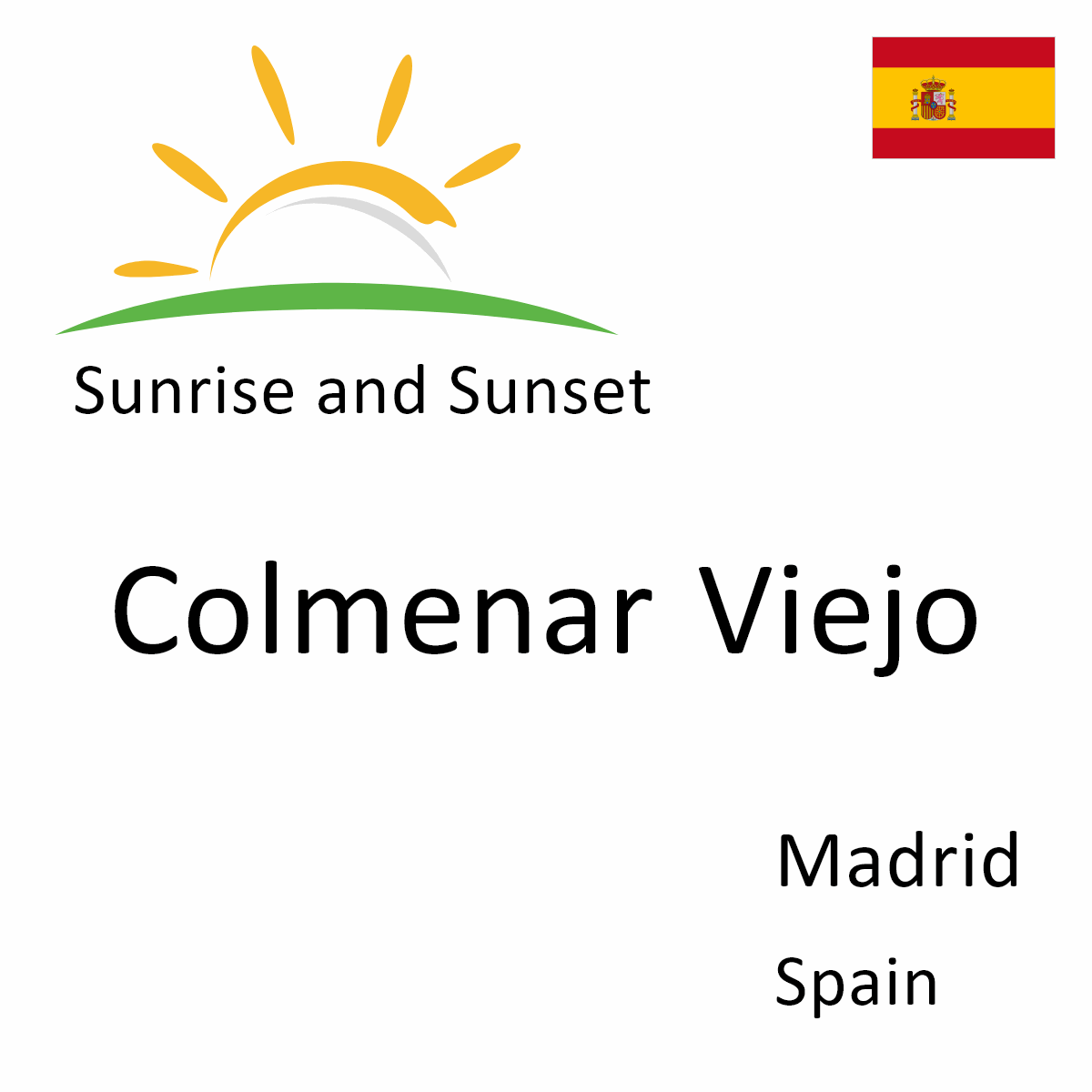The image features primarily text on a white backdrop with additional illustrations and elements. On the top left corner, there's a sketch of an abstract sun with radiating rays and a green horizon line, colored in yellow or possibly orange. The top right corner depicts a red and yellow striped flag, identified as the flag of Spain, with a wide yellow band across the center and narrower red bands above and below it. Along the top portion of the image, "sunrise and sunset" is written in black text. Centrally placed in slightly larger and bolder black letters is the name "Colmenar Viejo." Towards the bottom right, the text reads "Madrid" followed by "Spain."